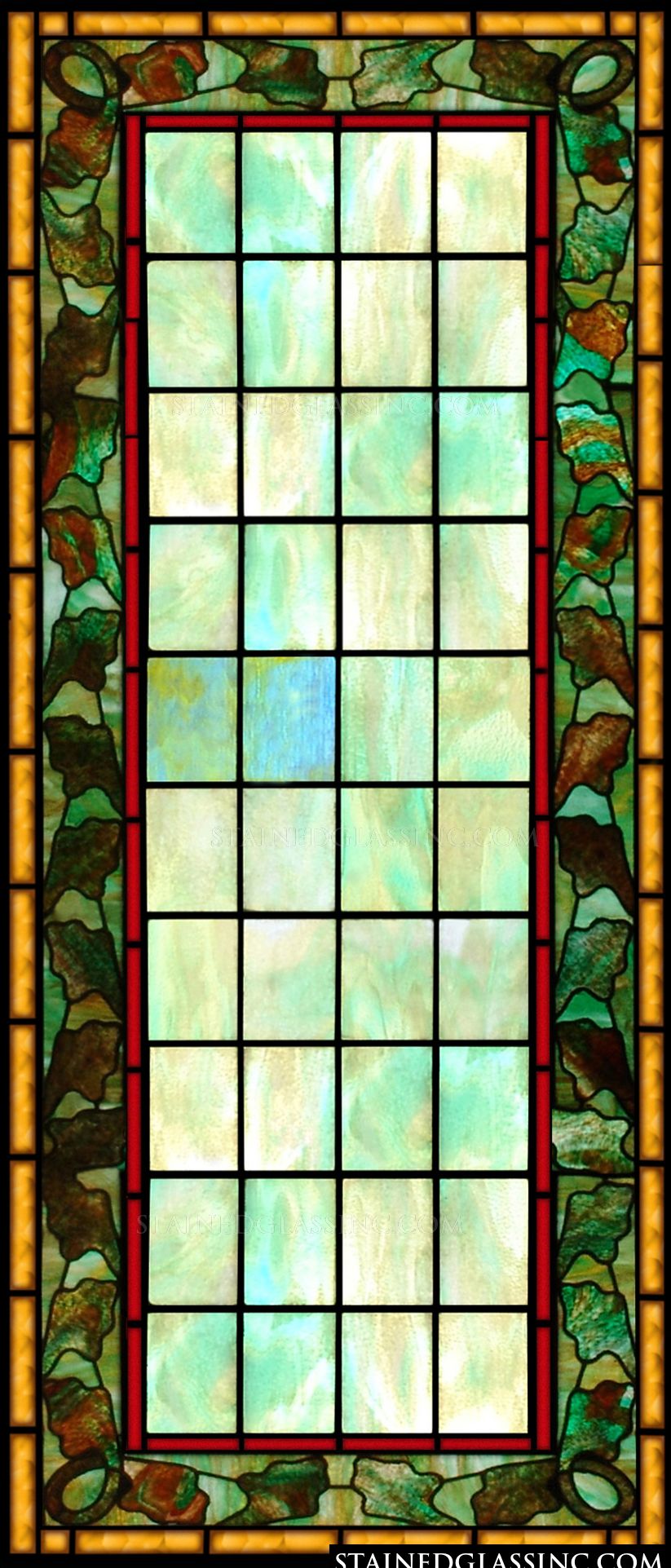The image showcases a tall, ornate stained glass panel that dominates the entire frame, set against a plain white background. The design appears to be well-suited for a door or a window, possibly found in places like a church or a mausoleum due to its classic and intricate design. The border of the panel features an orange-yellow frame, followed by a green frame representing leaves and vines, which are detailed with golden-yellow brickwork. Inside this border, a red rectangular frame encases a central area divided into smaller rectangles arranged in a 10 by 4 grid. These smaller panes are predominantly green with accents of yellow and blue. Additional colors within the design include shades of black, red, brown, and white, contributing to the piece's rich, colorful aesthetic. Text at the bottom right corner reads “stainedglassinc.com," indicating the likely manufacturer. The overall composition and alignment suggest a product image highlighting the detailed craftsmanship and elegant design of the stained glass panel.